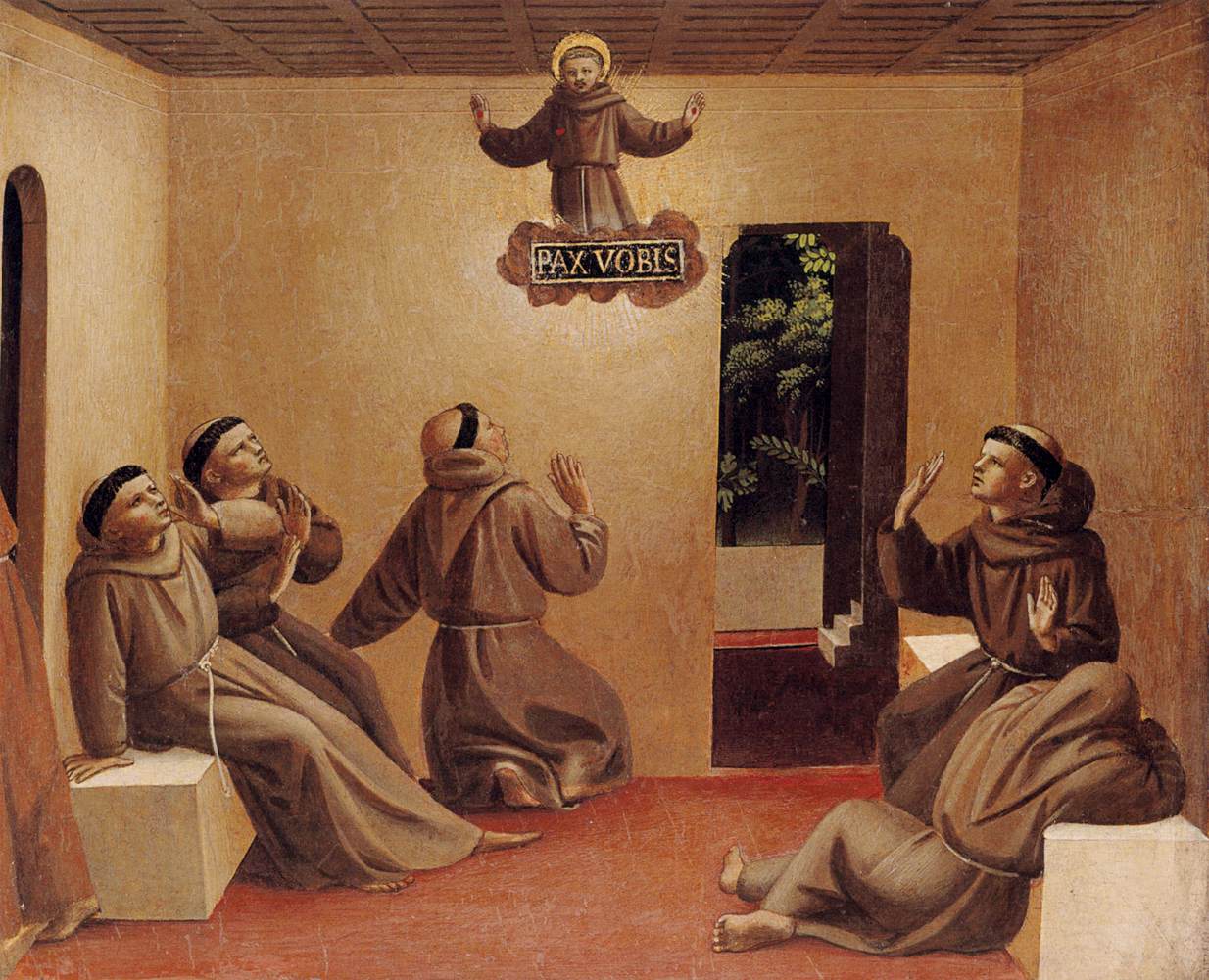In the painting "Apparition of St. Francis at Arles" by Fra Angelico, created in 1429, a profound religious scene is depicted. The room's red-painted floor contrasts with its tan walls and wooden or tiled ceiling. White marble benches line the sides. At the center is a deity, Saint Francis, adorned with a yellow halo, cloaked in long brown religious garb. Beneath him, the Latin inscription "PAX VOBIS" translates to "Peace be with you." 

Five youthful monks, either teenagers or in their early 20s, are dressed similarly in long, brown robes with sashes. Four monks gaze upwards with their hands raised towards Saint Francis, black headbands circling their tonsured heads. One monk kneels with an extended arm, two sit on a bench in reverence, and another, depicted with his hands lifted and palms showing, sits against the wall. In the corner, one monk, hood drawn, is draped over the bench with his face down. 

The room features two exits: a door to the right leading outside with greenery visible and another to the left where a sixth figure is departing. This image encapsulates a moment of divine encounter and spiritual devotion.